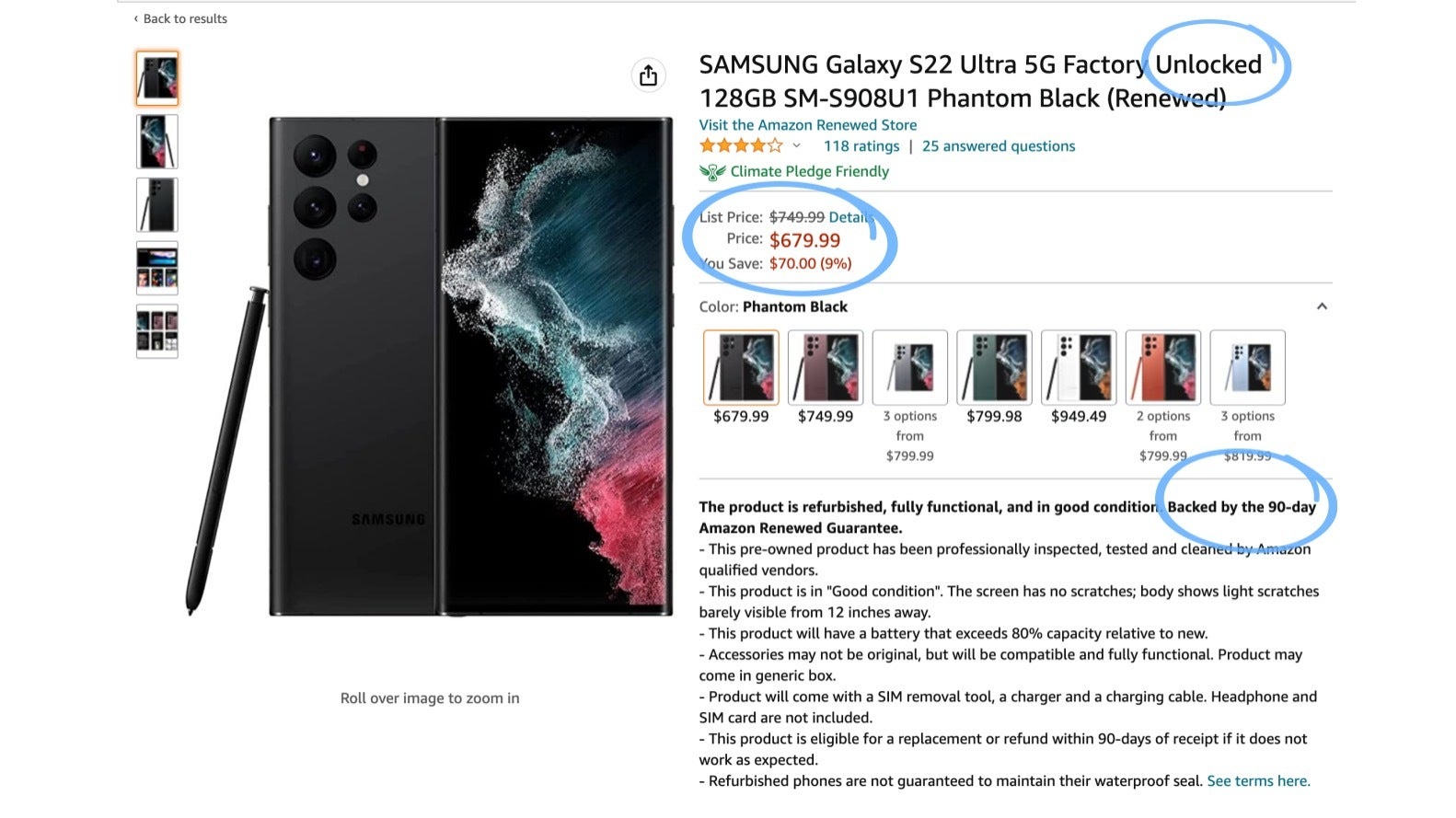This computer screenshot displays an online product listing for a Samsung Galaxy S22 Ultra 5G Factory Unlocked 128GB SM-S908U1 in Phantom Black, marked as 'renewed'. At the top, a gray horizontal navigation bar spans the width of the screen, with a small "Back to Results" link located in the upper left corner. Below, a vertical column on the left side showcases five unclear images, possibly of a tablet. The first image appears to be the back of a tablet device.

To the right of this vertical column is a larger, clearer image likely featuring the Samsung Galaxy S22 Ultra. This image is split into two sections: the left half is gray, the right half is black, and it displays a vibrant, multicolored wave that transitions from blue-green at the top to hot pink at the bottom. Along the top left edge of the gray section, three black circles are vertically aligned. Adjacent to them, on the right, are a black circle, a white circle, and another black circle. A gray stylus leans against the left side of this section.

Further to the right, the product description is prominently displayed in black text. It reads: "Samsung Galaxy S22 Ultra 5G Factory Unlocked 128GB SM-S908U1 Phantom Black (renewed)." The price sits below this description. Additional images showcasing the product in different views and colors are positioned beneath the primary details. At the bottom of the screenshot, several lines of fine print are visible in black text.